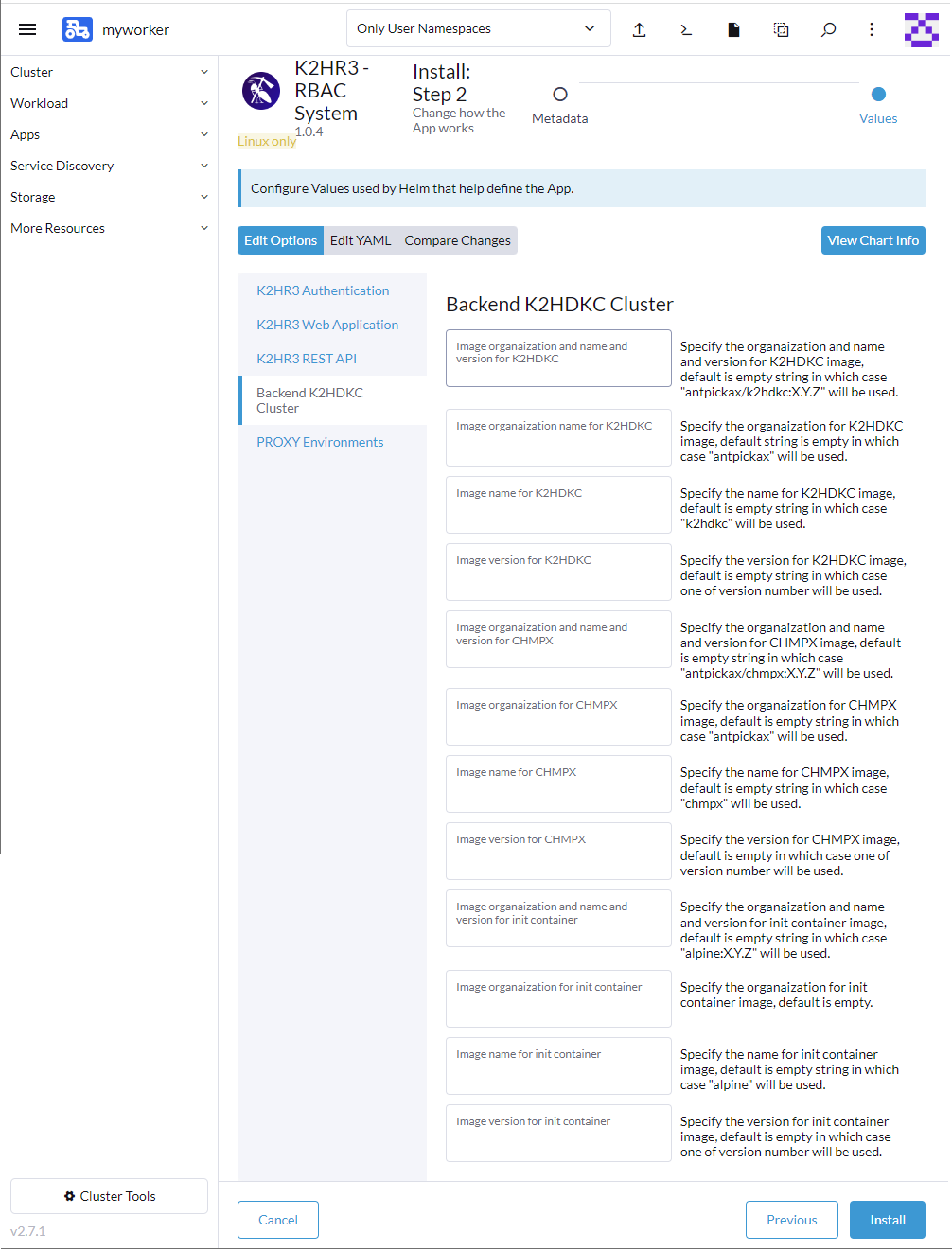The image appears to be a screenshot from a web-based tool, likely designed for administrative or data management purposes, possibly akin to a cluster control panel or a knowledge base interface such as Spiceworks. The interface has a clean, white background with information presented in various columns for ease of navigation and data interpretation. The layout features a left-side menu and a top menu adorned with icons, enhancing accessibility to different functionalities. The primary content area is split into multiple columns; one column appears to display overall search results, while another is bifurcated into a detailed breakdown or definition list of entries. This structured, data-driven layout suggests a focus on simplifying the user experience for managing or retrieving information efficiently.